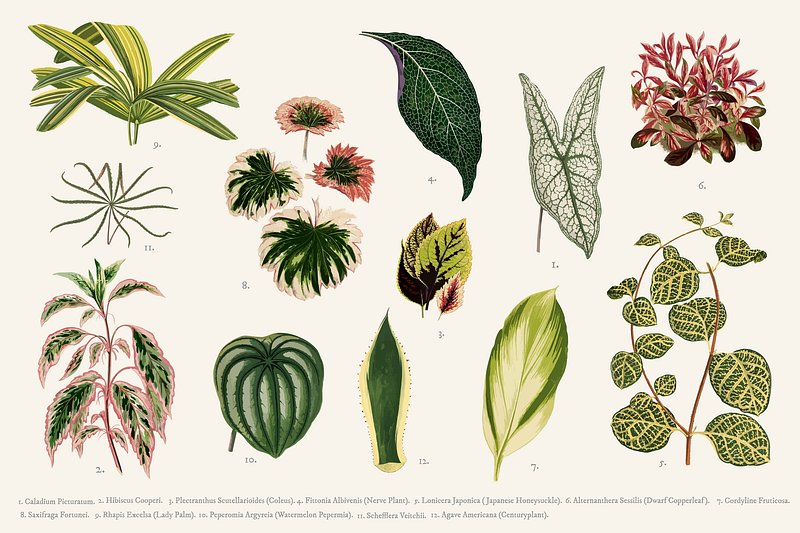The image showcases a scientific depiction of eleven diverse plant species, each meticulously illustrated on slightly yellowed, cream-colored paper suggestive of an old book page. The background's subtle off-white tone complements the detailed, colored drawings of the plants, emphasizing variegated leaves in shades of yellow, white, pale green, and dark green along with light pink flowers.

The plants are labeled with small textual identifiers, likely their genus and species names in black font, written in Latin and positioned at the bottom of the image. From left to right and top to bottom, the plants are arranged in a structured format. Notably, at the top left, there's an agave plant and below it, a spider plant. Adjacent plants include dark and light green leaves, and what appears to be a small green bush with hints of darker shades within its foliage. 

Further down, there's a vine-like plant leading to another with muted, greenish flowers. Additional varieties feature mint-like leaves, a large plant with striking dark green spots, a green melon-shaped plant, and others with unique leaf patterns, including a plant with a dark green backdrop and light green polka dots.

Overall, the image serves as an informative botanical chart, showcasing various plant species with an emphasis on their distinctive features and color variations.